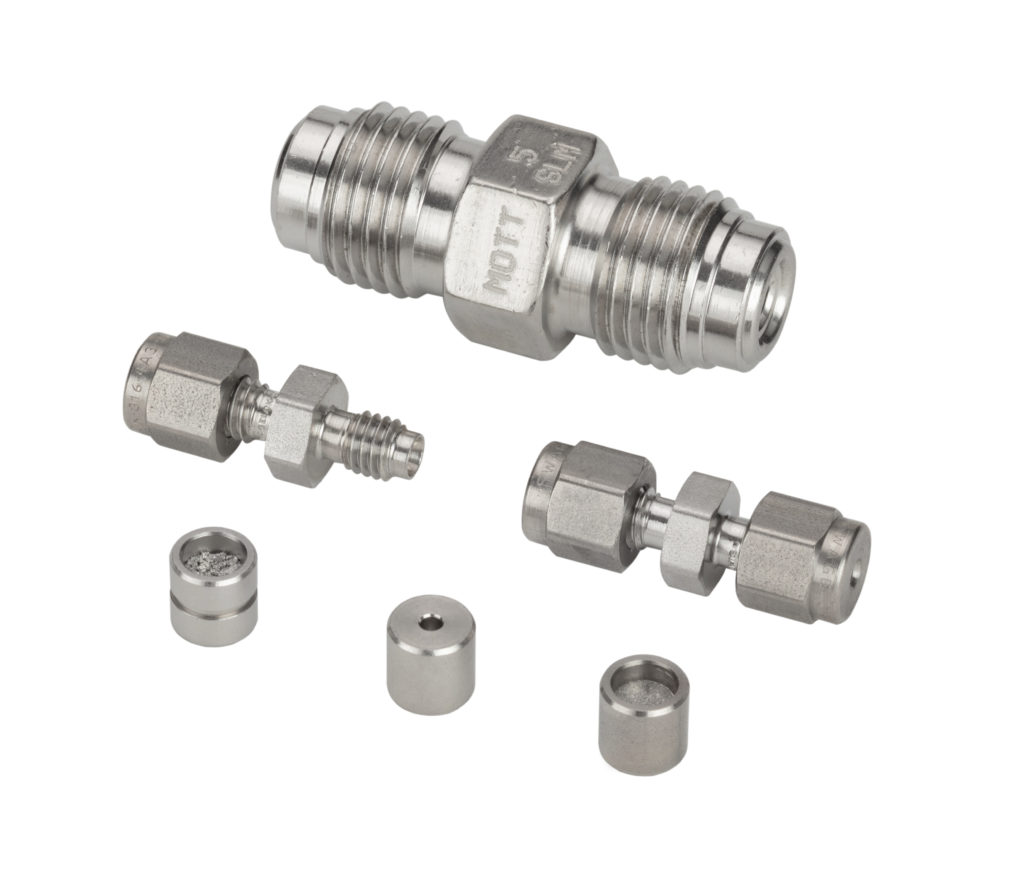The image showcases a set of metallic hardware components arranged against a clean, white background. At the top, there is a significantly larger piece, prominently displaying the brand name "MOTT" and some indistinct alphanumeric markings. This large piece has a central bar that extends out into pointed ends, resembling a bolt with threading.

Below this top piece are two sizeable silver components, each characterized by hexagonal shapes and threaded, screw-like ends. The one on the left features a large central unit with ridged edges and additional elements attached to its base, while the one on the right mirrors this structure with symmetrical, possibly detachable parts on both ends and a central section with ridges.

At the bottom, there are three smaller, oval-shaped items that appear to be nuts, completing the assembly depiction. These components collectively convey an array of mechanical elements, highlighting their screw ends and interlocking features, all meticulously positioned in the frame.